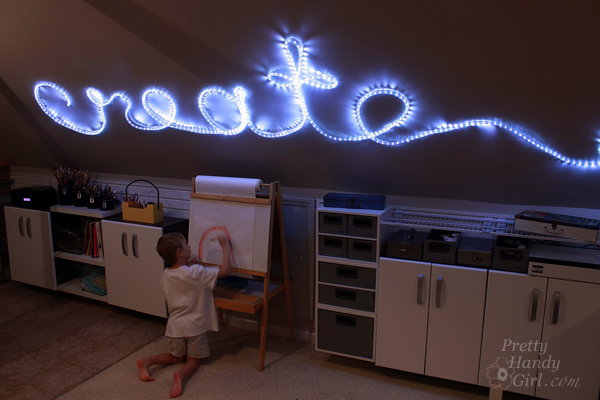The image captures a small boy, dressed in a white shirt and beige shorts, intently drawing with a red marker on a large sheet of white paper, which is mounted on an easel or board. He is kneeling in a room that appears to be a creative space or a child's playroom, characterized by a slanted ceiling and a range of cabinets and shelves along the wall. The left side of the room features cabinets with closed doors and a collection of cups filled with colored pencils atop them, indicative of ample art supplies. The cabinets and storage boxes, in shades of gray and white, contribute to the room's organized yet playful atmosphere. Overhead, a strip of light, fashioned into the word "create" in a flowy design, adorns the ceiling, enhancing the room's artistic ambiance. The photograph bears the watermark "prettyhandygirl.com" with a small flower illustration at the bottom right corner, suggesting the possible source or inspiration for the creative setting. The overall scene is one filled with the promise of creativity and imagination, ideal for nurturing a child's artistic endeavors.